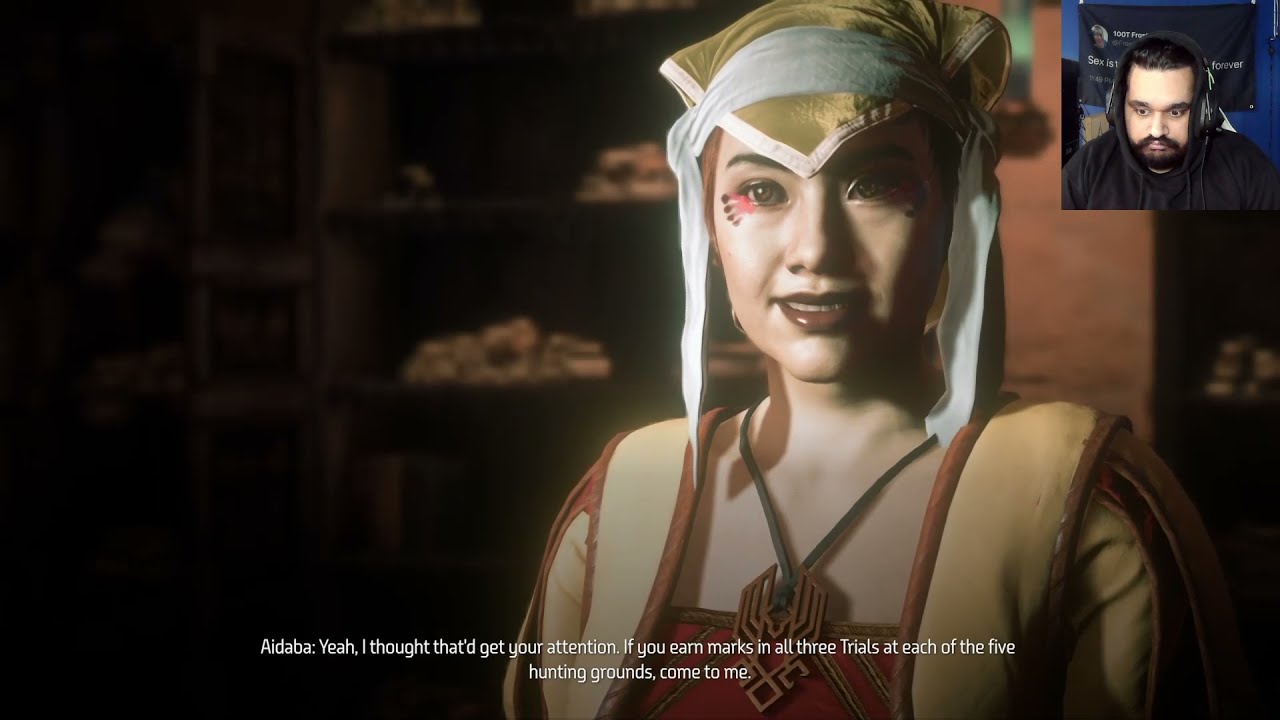The image depicts a highly detailed and lifelike character, possibly from a video game or movie, with a futuristic aesthetic reminiscent of Dune or Star Wars. Central to the image is an Asian woman adorned in elaborate attire, including a gold headdress with white scarf-like flaps and an intricate necklace or amulet. Her makeup features bold pink eyeshadow with black and red paint accentuating her right eye, which is the only one visible due to the shadows enveloping the rest of her face. She wears a luxurious gold and red gown with a red top. In the background, there's a shadowy area with what appears to be cupboards and shelves, making it difficult to discern finer details.

In the upper right-hand corner, a man with a mustache, beard, and black hair is visible. He wears headphones and a hooded jacket, almost blending in but distinguished by his lifelike features that leave one questioning whether he is a photograph or an avatar. The bottom of the image contains white text that reads, "Adaba: I thought that'd get your attention. If you earn marks in all three trials at each of the five hunting grounds, come to me," further suggesting a narrative or mission related to a game. The general blue tint in the background adds to the immersive and possibly digital environment of the scene.